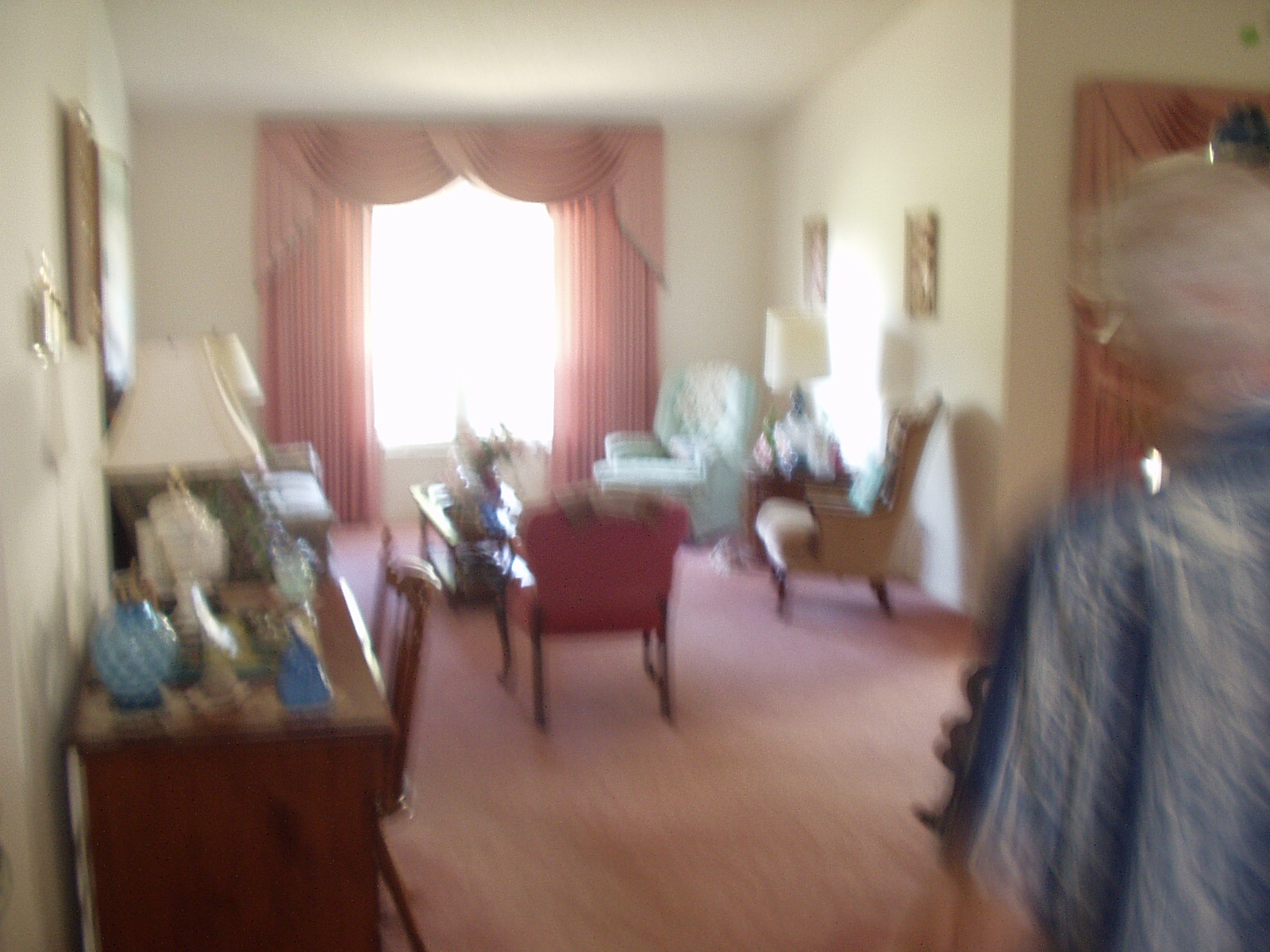The image is quite blurry and out of focus, capturing a modest, well-lived-in living room, likely belonging to an older person. The room is warmly decorated with pink curtains that have a cascading valance draped over the top, adding a touch of elegance. To the left, there are two framed photographs hanging on the wall. Below the frames, a small end table stands, adorned with a lamp and various tchotchkes.

In the background, a blue armchair occupies the back corner, creating a cozy nook. Adjacent to the end table on the right is a brown sitting chair, likely used for relaxation or reading. The center of the room is defined by a wooden coffee table, which serves as a focal point amidst the furniture.

Another seating option, a burgundy armchair, is positioned in the center of the photo with its back facing the viewer. In the bottom left corner, a wooden desk complete with a matching chair hosts a lamp and other decorative items on top, suggesting it might be a space for writing or hobbies.

Adding to the homely atmosphere, the room features a pink carpet, which coordinates with the curtains. On the left edge of the photograph, part of the back of a person with white hair dressed in a blue dress is visible, further indicating this space is lived-in and cherished.